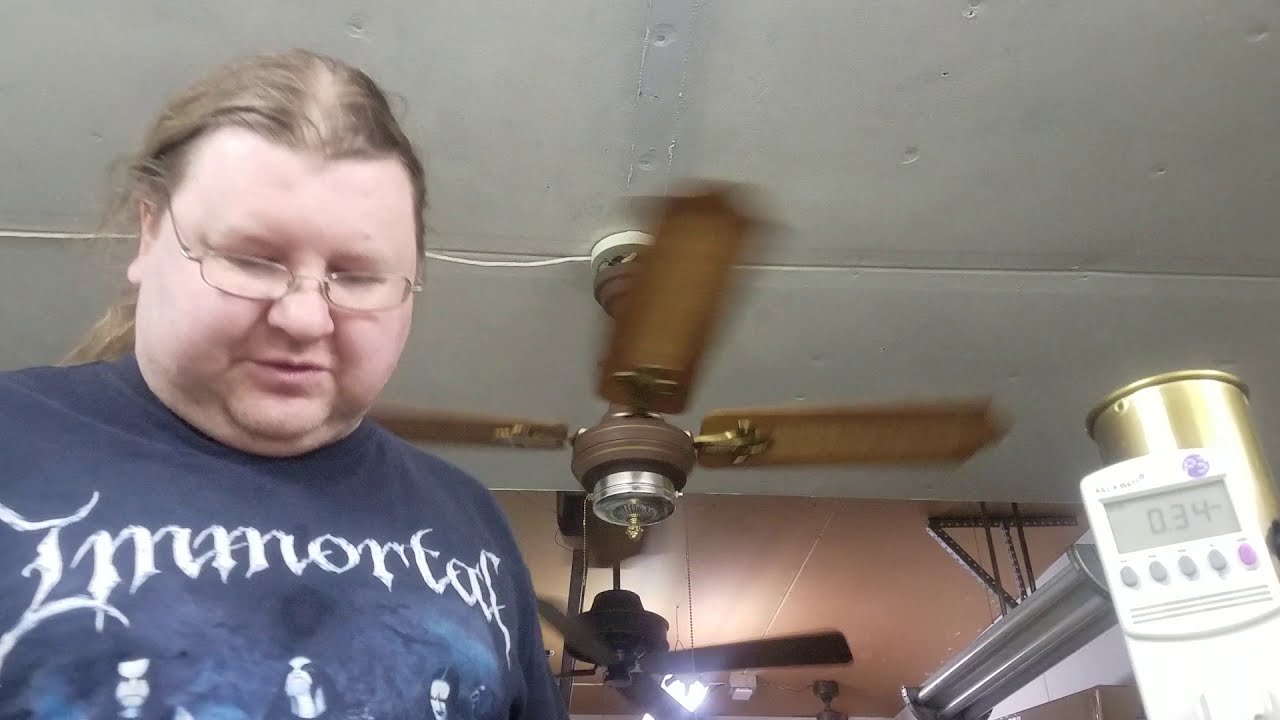This indoor image features a slightly overweight Caucasian male with long, dirty blonde hair tied back in a ponytail. He is wearing thin-framed glasses and a light gray t-shirt with the word "Immortal" emblazoned in white letters. The t-shirt also depicts three men with face makeup and long dark hair, resembling members of a metal band. The man appears to be looking downwards, with his eyes closed or partially closed. In the background, there are two ceiling fans mounted on the white ceiling, one of which appears to be in motion. To the bottom right corner of the image, a device with a screen displaying "0.34" and several buttons is visible, likely some kind of thermostat or mechanical device.